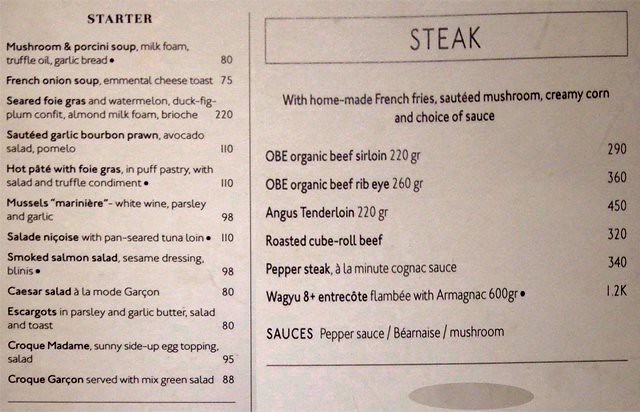The image depicts a light brown, cream-colored restaurant menu divided into two columns by a thin vertical black line. The left side is labeled "STARTER" and offers a detailed list of appetizers along with their prices. These include Mushroom and Porcini Soup ($80), French Onion Soup ($75), Seared Foie Gras, Sautéed Garlic Bourbon Prawns, Hot Pâté with Foie Gras, Mussels Marinara, Salade Niçoise, Smoked Salmon Salad, Caesar Salad, Escargot, Croque Madame, and Croque Garcon. The right side is dedicated to the main course, highlighted by the heading "STEAK" written within a rectangle. Below, it clarifies that all steak options come with homemade French fries, sautéed mushrooms, creamy corn, and a choice of sauce. The menu lists various types of steak, including Angus Tenderloin, Roasted Cube Roll Beef, Pepper Steak, and Wagyu, along with their respective weights and prices.